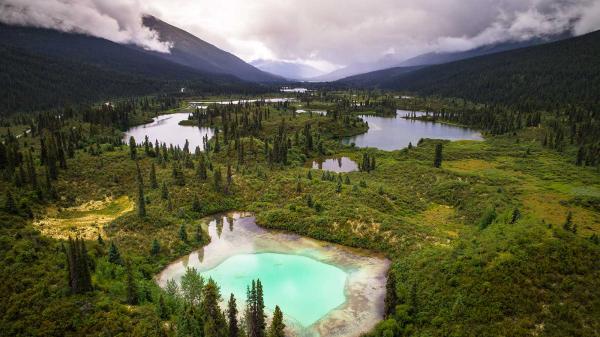This photograph captures a stunning natural landscape, likely snapped from an aerial perspective, showcasing a serene valley nestled between two majestic mountains. The mountains, painted in hues of purple and blue, slowly rise from a central point, their peaks shrouded in a rolling blanket of clouds. The sky above is mostly gray with a hint of sunlight peeking through in the background. The valley floor is lush with greenery, dotted with scrubby, baby trees and pointy, conical foliage that testify to the untouched, natural beauty of the area.

Prominently featured in the foreground is a striking turquoise blue pool of water, surrounded by sandy terrain, serving as the focal point of the image. This unique pool, along with several other smaller bodies of water that seem to spread out down the valley, appears as bright, reflective patches amidst the green flatland. These natural pools, forming what looks to be part of a larger swampy region, are interspersed with areas where it's unclear if the greenery is solid ground or vegetation on water, enhancing the mysterious allure of the landscape. The overall ambiance of the scene is peaceful and quiet, devoid of any visible wildlife or human presence, making it a truly scenic and untouched natural haven.